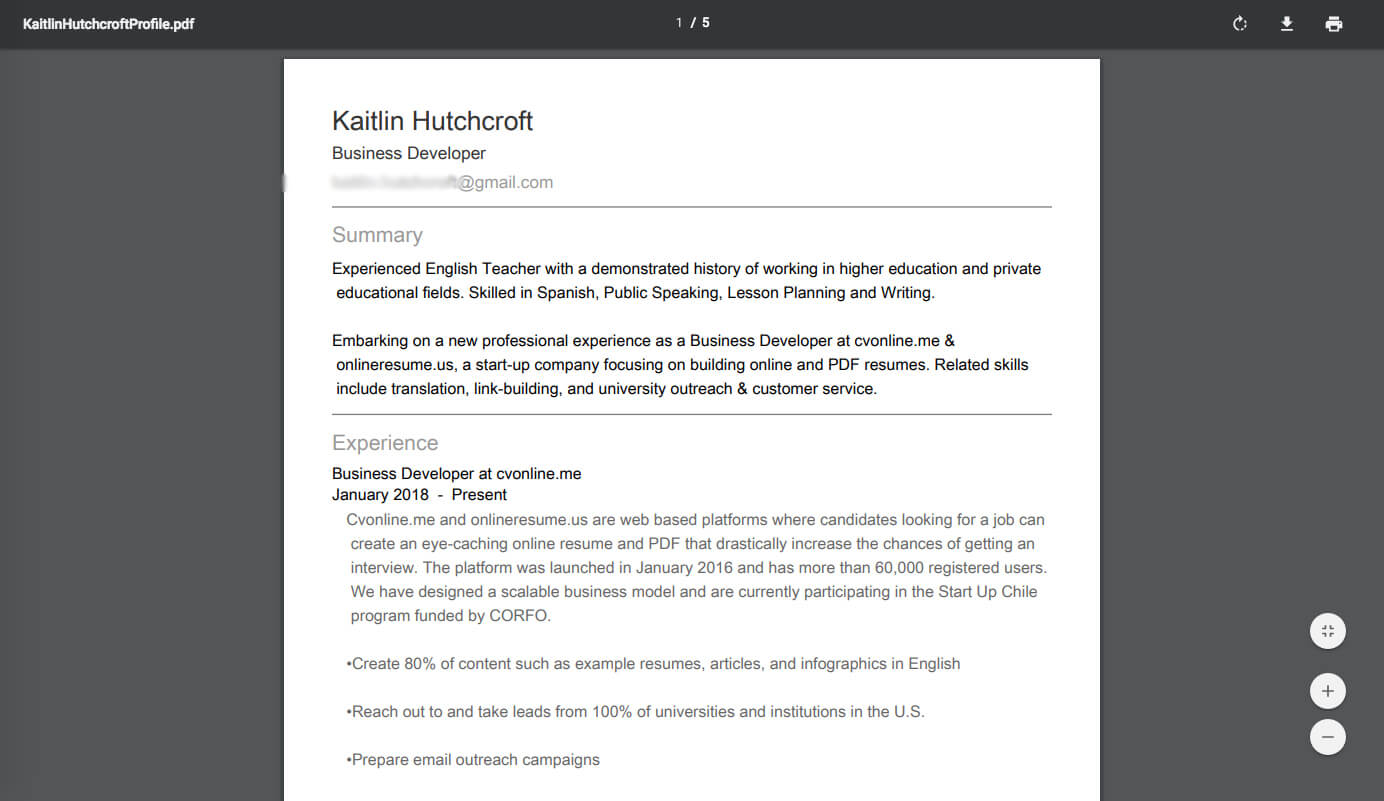The image depicts what appears to be the first page of Caitlin Hutchcroft's resume, formatted as Caitlin_Hutchcroft_profile.pdf. The document, likely created on a computer, shows various icons for printing, downloading, and returning to a previous page.

At the top of the document, the header prominently displays "Caitlin Hutchcroft, Business Developer," alongside a blurred-out email address to protect privacy. Below the header is a professional summary, which highlights Caitlin's background as an experienced English teacher with a proven track record in higher education and private educational fields. The summary further notes her skills in Spanish, public speaking, lesson planning, and writing.

The next section details Caitlin's career transition, stating, "Embarking on a new professional experience as a Business Developer at cvonline.me and onlineresume.us, a startup company focusing on building online and PDF resumes." This paragraph also outlines her relevant skills including translation, link building, university outreach, and customer service.

Following the summary, the resume lists Caitlin's professional experience, beginning with her most recent role from January 2018 to the present. This section includes a brief paragraph describing her responsibilities and achievements, supplemented by three concise bullet points that provide further detail.

Overall, the document provides a clear picture of Caitlin Hutchcroft's professional experience and skill set.